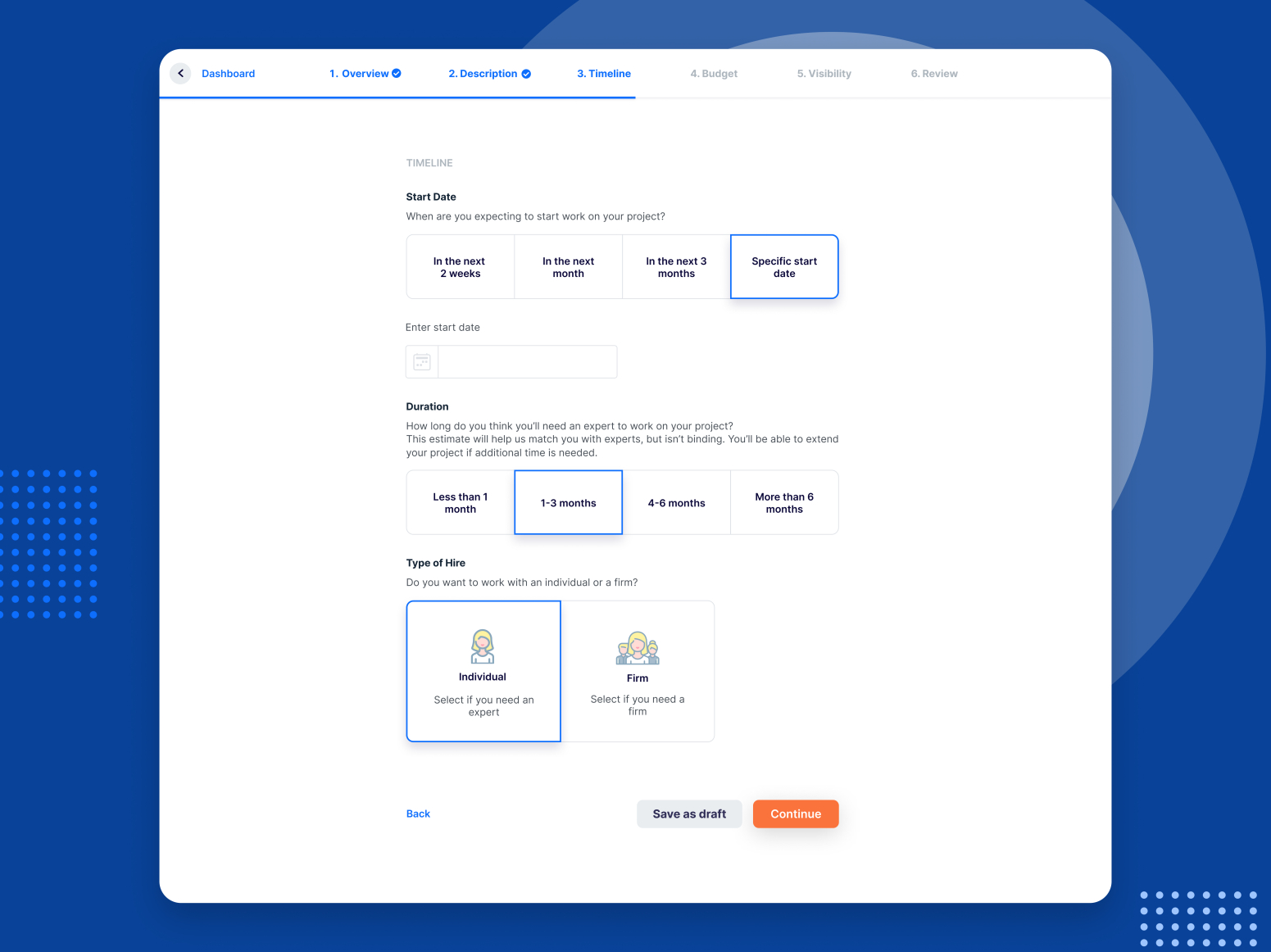This image appears to be a screenshot of a project management dashboard on a website. The interface shows multiple tabs open along the top, with a navigational arrow in the upper left corner labeled "Dashboard." The various tabs are sequentially numbered one through six, each representing different stages or sections of the project setup. The first tab, labeled "Overview," and the second tab, labeled "Description," have been checked off, indicating their completion. The current active tab is "Timeline," which is followed by tabs for "Budget," "Visibility," and "Review."

Within the "Timeline" tab, several prompts and options are visible. It asks, "When are you expecting to start work on your project?" with multiple choices provided, including an option to enter an exact start date. Another section titled "Duration" asks, "How long do you think you'll need an expert for the project?" where users can specify a time frame. Additionally, it inquires about the "Type of hire," prompting users to choose between working with an individual or a firm. At the bottom of this section, there are options to either "Save as Draft" or "Continue" to the next step in the project setup process.